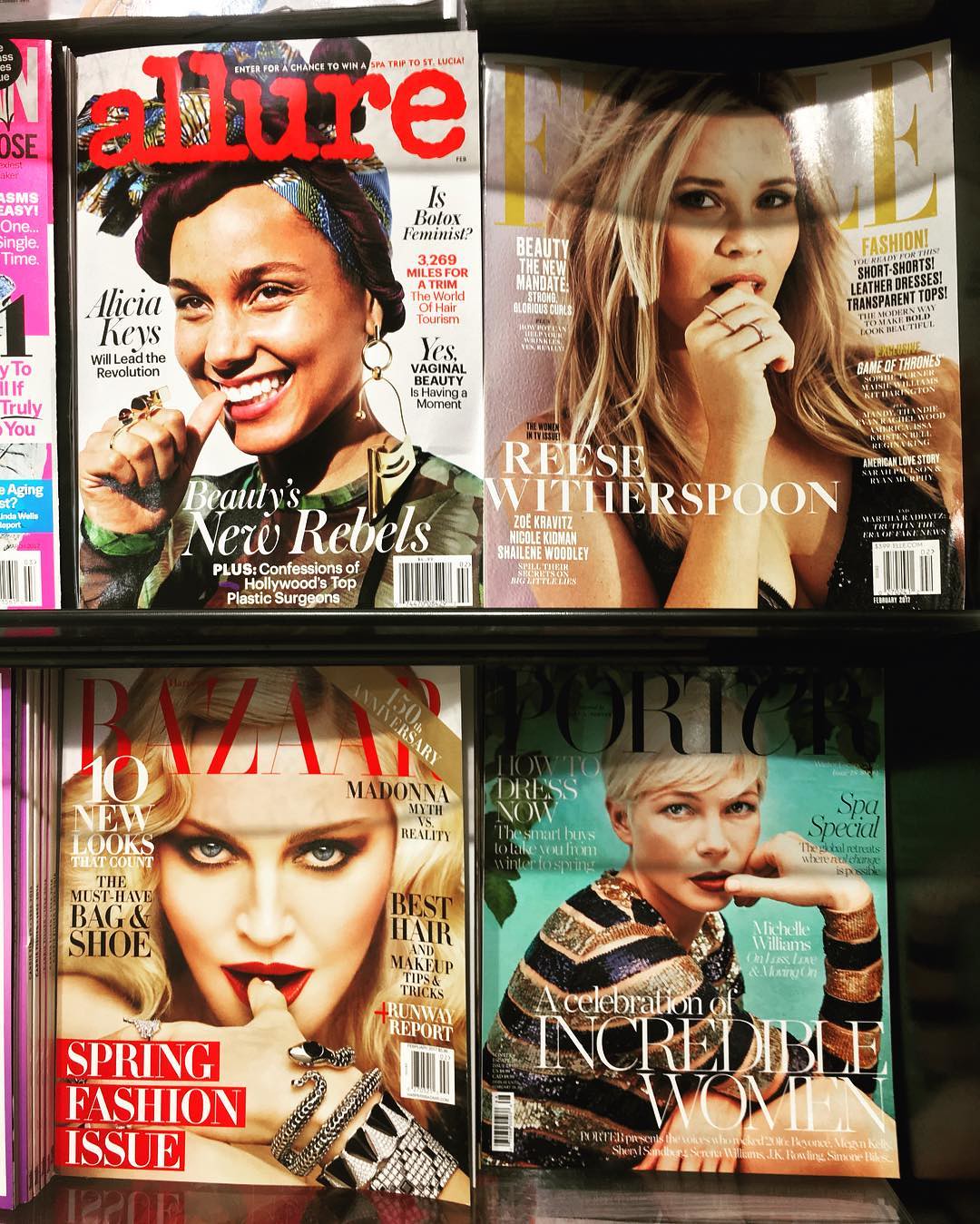The photograph captures a magazine stand with two black shelves loaded with fashion magazines, each featuring prominent women on the covers. On the top left shelf, there's an Allure magazine showcasing Alicia Keys in a white blouse with a hairband, smiling with her thumb near her mouth. Adjacent to it on the top right is an Elle magazine featuring Reese Witherspoon with a seductive look and her thumb also near her mouth. The bottom left shelf holds a Bazaar magazine, a spring fashion issue with Madonna on the cover, similarly posing with her thumb towards her mouth. The bottom right magazine has a name that's not fully clear, possibly "Lori" or "Portico," and features a blonde woman, likely Michelle Williams, wearing a striped blouse with short blonde hair and a pensive look, her hand resting on her cheek. All four magazines emphasize powerful women, each uniquely styled yet sharing the common theme of having their thumbs near their mouths.